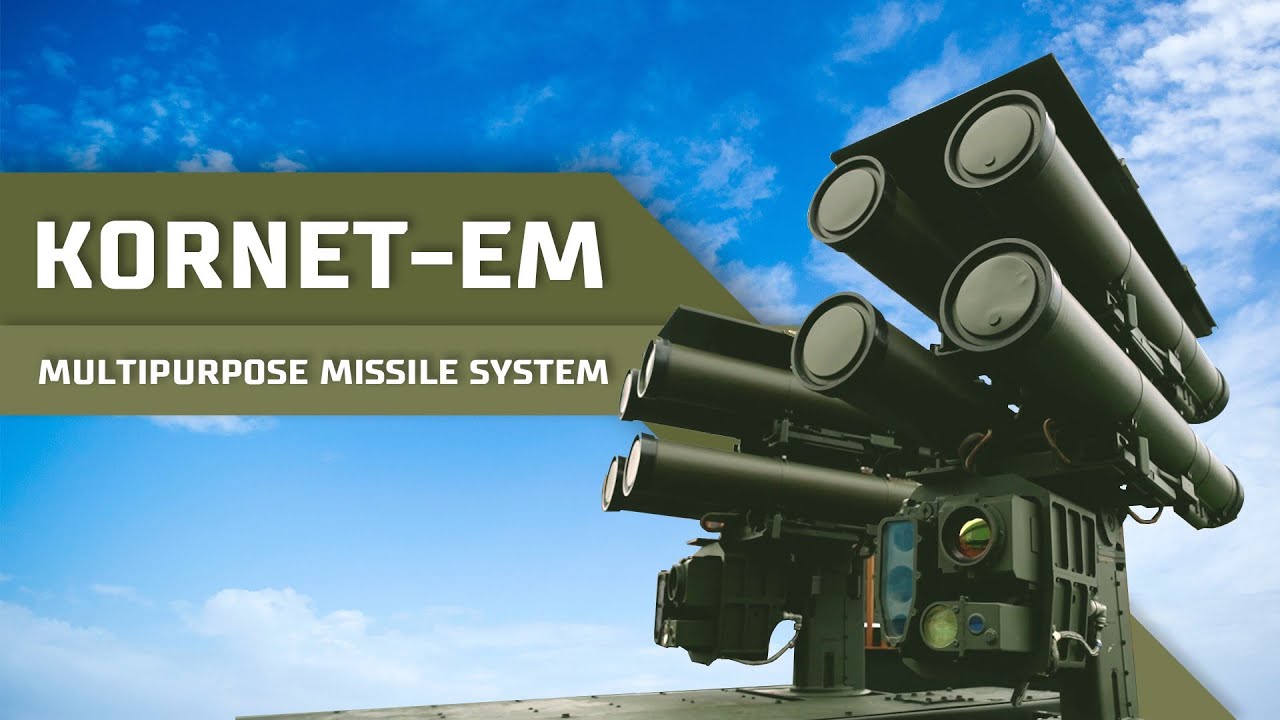The image features an advertisement for the Cornet-M multi-purpose missile system, and showcases a sophisticated piece of military equipment against a serene sky backdrop. The prominent Cornet-M logo is positioned to the left, highlighted by a forest green background that echoes traditional army colors. The missile system, which appears mounted for potential use on a vehicle like a tank, stands off-centered to the right and features eight visible tubular rocket launchers. Below these launchers, there's an assembly that includes what looks like a video recording device, multiple lenses, and possibly a light for nighttime operations. The overall aesthetic and design clearly indicate its intended military or law enforcement applications.